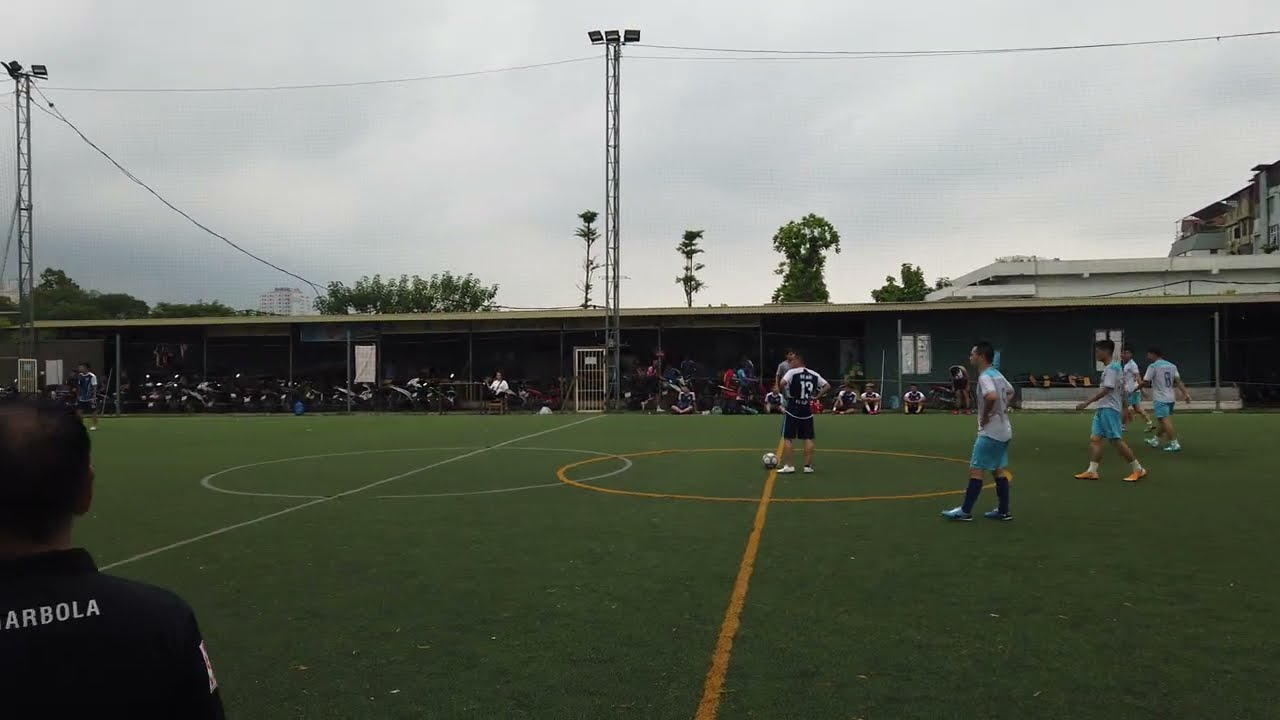This image captures an outdoor scene on what appears to be a football field, though it might be mistaken for a soccer field due to the setup. In the foreground, the green, grass-covered field is clearly marked with white and yellow lines, including circular markings, typical of sports fields. A football (or possibly a soccer ball) is placed at the center of the field. To the left, a coach stands with his back to the camera, wearing a jacket adorned with white letters. Players dressed in various uniforms—some in black and white, others in white and light blue—are positioned at the far edge of the field, seemingly preparing for the game.

On the right-hand side, additional players and some vehicles are visible. In the background, a flat building spans the width of the image, possibly serving as a dugout or a place for spectators. Several people are seated or standing in sections of this building, watching the scene on the field. Beyond this structure, a line of trees and tall, metallic light towers stretch towards the sky, which is partly obscured by gray clouds, indicating an overcast day.